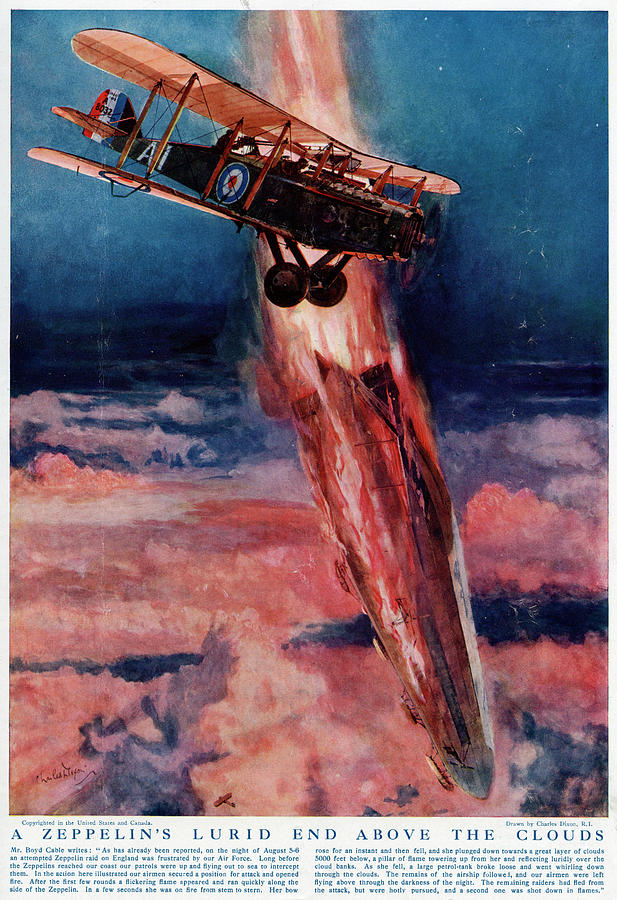The detailed illustration, reminiscent of an old magazine cover, vividly depicts a dramatic aerial scene from the 1920s. In the foreground, a red biplane with British RAF insignias—distinguished by blue, white, and red bullseye markings—is soaring to the right. Its propeller spins, and its tail fin is marked with the iconic red, white, and blue stripes. Below it, a large Zeppelin, cylindrical and shrouded in smoke, plummets from the sky, suggesting a chaotic aerial battle. Above this perilous descent, a comet streaks through the blue sky, its fiery tail blazing towards a white-hot tip, adding to the scene's sense of urgency and danger. The entire image is bathed in a reddish hue, creating an ominous atmosphere, with clouds at the bottom tinged in reddish-pink, seemingly scorched by the destruction unfolding above. At the very bottom, a text layer occupies about 15% of the composition, displaying a headline in black ink that reads, "A Zeppelin's Lurid and Above the Clouds." This is followed by an article snippet starting with, "Mr. Boyd Cable writes, as has already been reported on the night of August 5-6, an attempted Zeppelin raid on England was frustrated by our Air Force," hinting at the historical context of the scene.